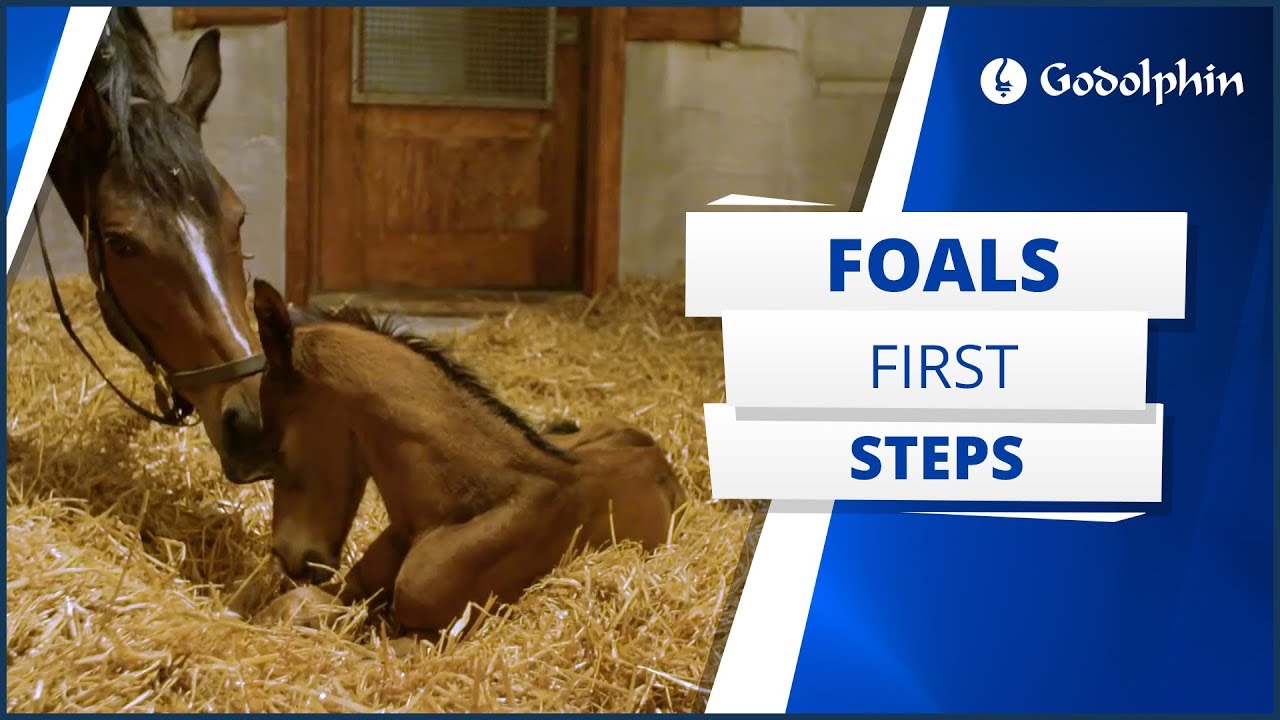A security camera screenshot captures the touching moment between a brown mare and her newborn foal, lying on a bed of hay inside a stable. The larger horse, identified by a distinctive white stripe down the center of its face and wearing a bridle, gently pets the foal with its head from the upper left corner of the frame. The foal, still lying down as it has just been born, is enveloped in the golden hay spread across the stable floor. The stable itself features a wooden door with what appear to be blinds, and the background includes a concrete wall with a light gray tone and a blue gradient overlay with white diagonal stripes. White text at the top of the screenshot reads "Foals First Steps" within three rectangular boxes, accompanied by the Godolphin logo, which is a circular symbol, in the upper right corner.